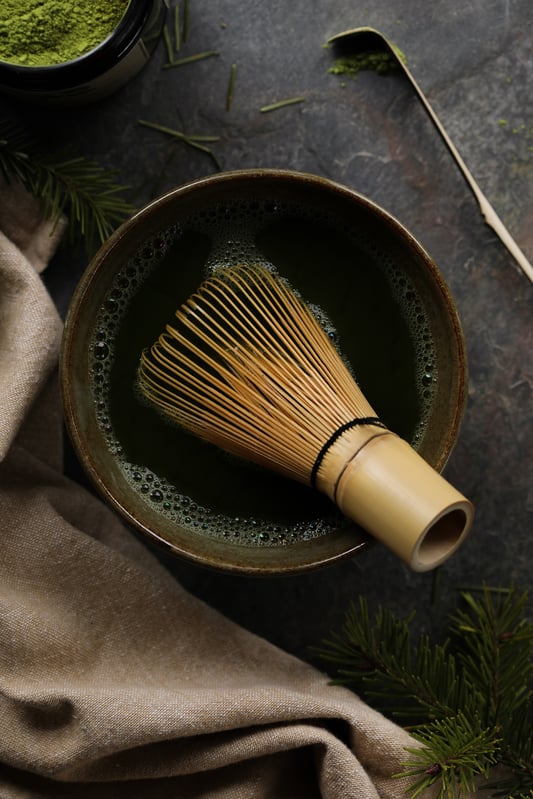An overhead, professionally staged shot features a dark, possibly clay, bowl sitting on a stony, dark granite or marble countertop. Inside the bowl, a unique wooden whisk with a stout, hollow handle resembling the top of a wine bottle and tightly bunched goldish-orange metal wires is soaking in a darker liquid with bubbles around the rim. A straw-like bamboo strainer is also visible, suggesting the preparation of a traditional tea. Surrounding the bowl, there's a crumpled tan burlap sack and sprigs of spruce or fir in various positions. Additionally, there's a small tin of bright green powder, likely green tea, accompanied by a thin metal spoon-like utensil from an Asian tea set, with some powder sprinkled on the surface. The scene also includes a partially visible brown bowl containing green powder in the top left and a metallic utensil, possibly a fork or spoon, near the top of the image. This setup, ideal for Instagram or a food blog, exudes a rustic yet sophisticated tea preparation ambiance.